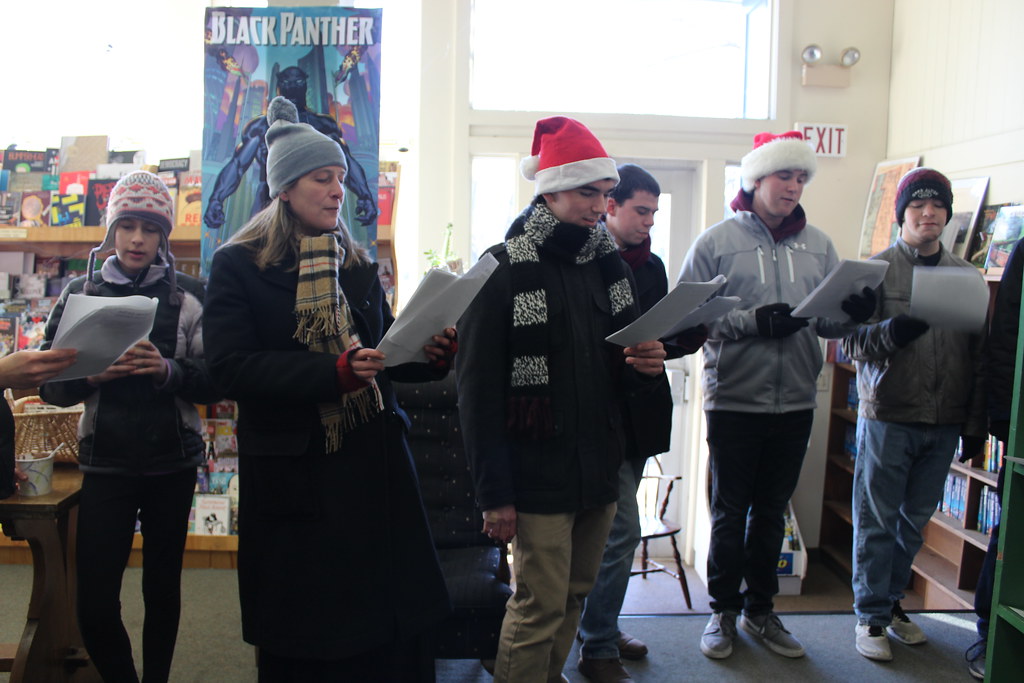The image captures a lively group of people in what appears to be a comic bookstore or library, evidenced by a rack of graphic novels or magazines visible in the background. Prominently displayed is a Black Panther banner, featuring the superhero T'Challa in his iconic catsuit with "Black Panther" written in white font. The setting is bright, with sunlight streaming through a doorway, though the crispness of the scene suggests it is winter. The group consists of six individuals, some standing on a raised platform while others remain on the ground. They are dressed warmly in coats, scarves, gloves, and Santa hats, indicative of the holiday season. Each person is holding stapled sheets of paper, seemingly engaged in singing or reading—a Christmas caroling activity is strongly implied by their concentrated looks and festive attire. The scene is set against a backdrop of cinder block walls, further grounding the festive snapshot in a cozy, indoor environment.